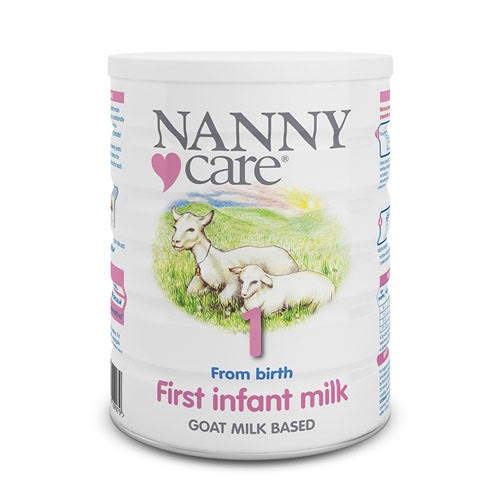In the image, there's a product displayed against a completely white background. The product is an off-white aluminum tin can labeled as "NANNY CARE," with "NANNY" in all caps on the first line and "care" in lowercase on the second line, preceded by a small pink heart icon. The can has a cylindrical shape with a lid on top. 

On the center of the can's label, there's a circular illustration featuring a pastoral scene: two goats, a mother goat with a red necklace, and an infant goat lie on a green grassland. The background of the illustration reveals hills, a blue sky with white clouds, and a yellow sun. Below the illustration, there are inscriptions in various colors. The number "1" is shown in pink, followed by "From Birth" written in blue text. Underneath, "FIRST INFANT MILK" appears in pink, and "GOAT MILK BASED" is written in black text. The composition is clean and serene, with hints of additional product details visible along the right and left edges of the can, including a barcode.